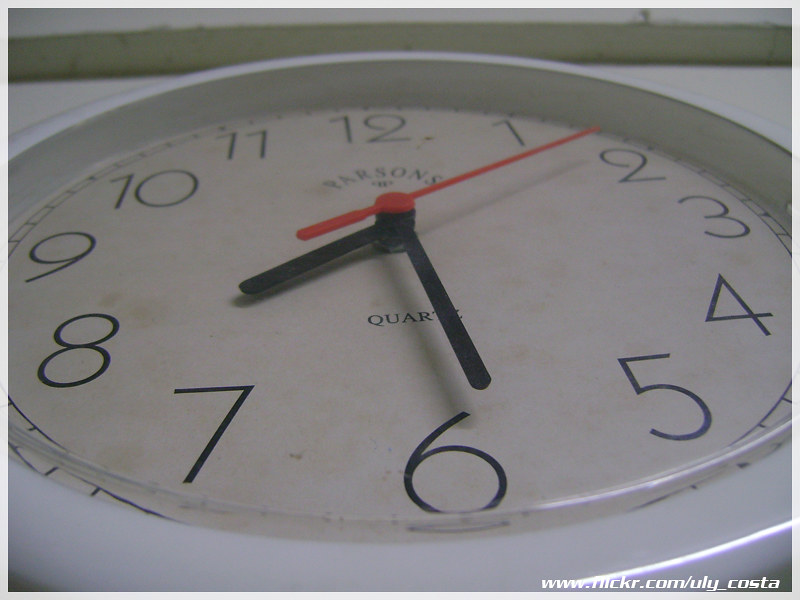This horizontal rectangular image features a large, seemingly vintage clock prominently displayed against a white surface, bordered by a thin, white frame and set against a green backdrop, possibly wood. The clock itself has a white or silver bezel surrounding its face, which is cream-colored, resembling ancient parchment. The dark-background image highlights the clock’s pristine exterior, with its white see-through glass or plastic cover adding a shiny touch. The clock face displays black, standard numerical digits and has three hands: black for the hour and minute, and red for the seconds. The current time reads approximately 7:30, with the red second hand between the one and the two. At the top of the clock face, "Parsons" is written in an arch shape, followed by "Quartz" underneath. Notably, in the bottom right corner of the image, there is white text that reads "www.flickr.com/uly_costa."